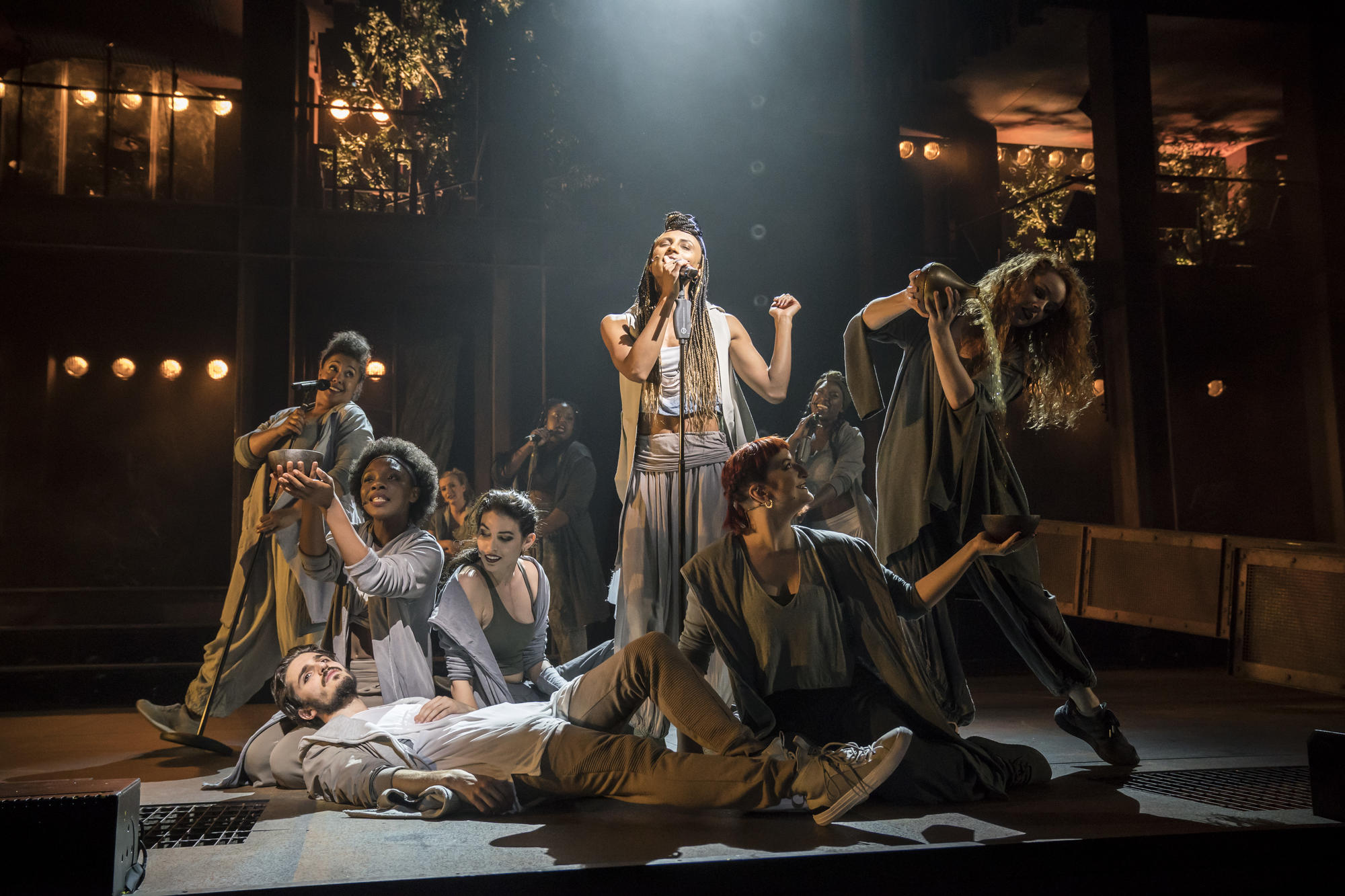In a dimly lit stage scene reminiscent of a small musical production, a female performer stands center stage, illuminated by a spotlight from above. She wears a drapey gray skirt and a sleeveless vest-like top over a white tank top, her eyes closed and head tilted back, seemingly lost in song. A microphone stands before her, amplifying her voice. A richly detailed backdrop, adorned with Victorian-style lights and a dark curtain, surrounds the performers. 

Around her, a diverse group of actors—some sitting, some standing—fill the scene. Three sit, one lounges on the floor, and several more stand nearby, also singing into microphones. One female actor pours water into a bowl held by another seated on the floor, creating a dynamic and engaging tableau. The performers, all clad in shades of gray and baggy garments that resemble a mix of hoodies, sweatpants, and possibly togas, contribute to the intimate, almost bohemian atmosphere. This evocative image portrays a cohesive ensemble, perhaps from a modern, gritty production like "Rent," united in a moment of theatrical expression against a backdrop of brown and yellow ambient lights that evoke the feel of an outdoor garden lit by string lights.